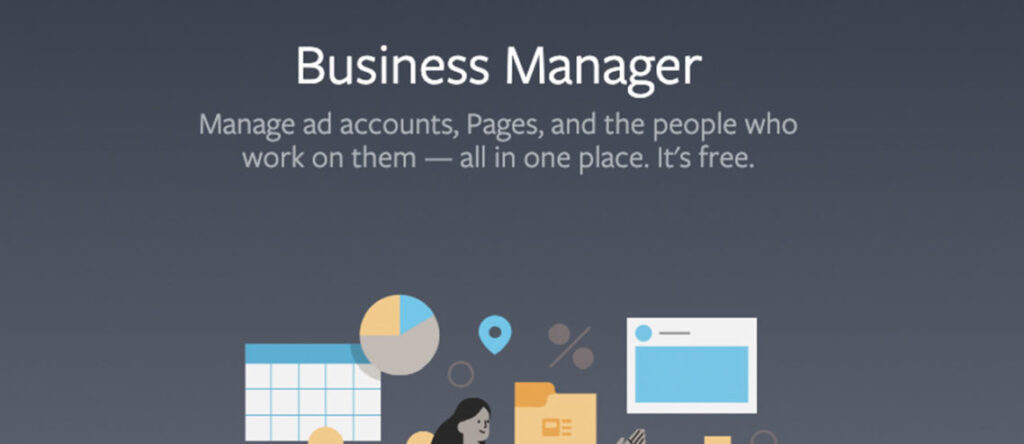This online banner features a dark grey background and prominently displays the text "Business Manager" in large, bold white font at the top center. Just below, in smaller grey lettering, it reads, "Manage ad accounts, pages, and the people who work on them all in one place. It's free." The design includes various cartoon images depicting business-related elements: several pie charts, calendar charts, and folders with tabs. A female character with black hair appears within the graphics, marked by a blue location dot above her head. Additional icons like a percentage sign and a transparent circle are also present. Although the banner is partially cut off at the bottom, the visible graphics suggest a continued theme of charts, office-related items, and mathematical symbols, emphasizing organizational tools and business management.